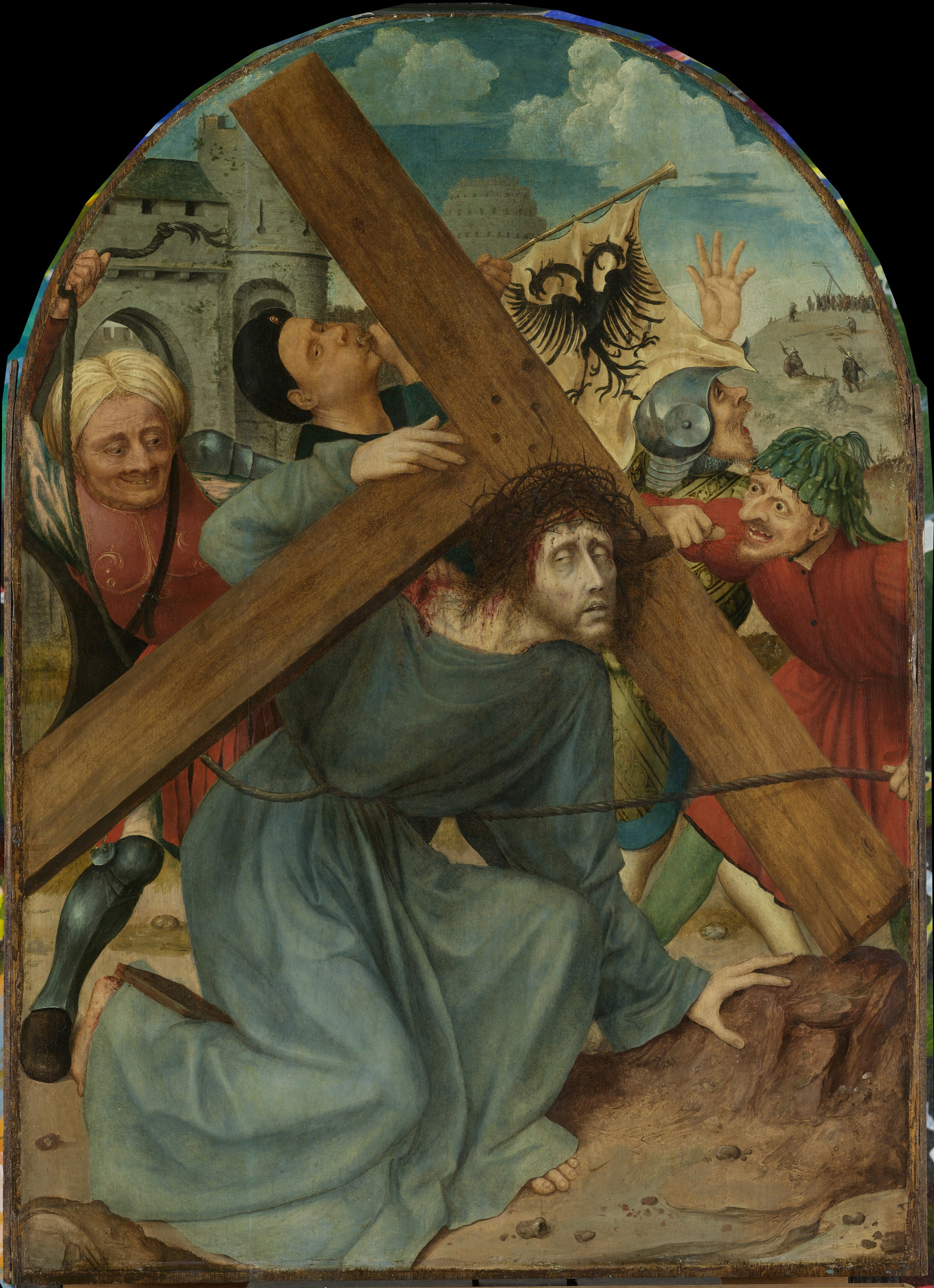This detailed image depicts a vibrant, arch-topped painting from biblical times featuring a scene of Jesus carrying the cross on his way to crucifixion. Positioned centrally, Jesus, with curly brown hair and a blue robe tied at the waist, is on one knee, gazing slightly to the right and upwards. His left hand rests on a rock at the bottom right of the frame. The wooden cross, borne on his back, enters the image from the left, extending up and to the right with the horizontal beam stretching both upwards to the left and downwards to the right.

Surrounding Jesus are several figures in traditional attire from the era. To his left stands a blonde-haired individual in a red tunic, casting a leer towards Jesus. On the right, another figure, donning a green cap and red robe, has a hand on the cross. Behind them, other spectators can be seen, one looking up with a hand on the cross. In the background on the left side, there's a gray structure or castle, while on the right, the landscape ascends into a hill under a blue sky decorated with clouds. The scene's contextual details evoke the visual storytelling style reminiscent of old religious films.